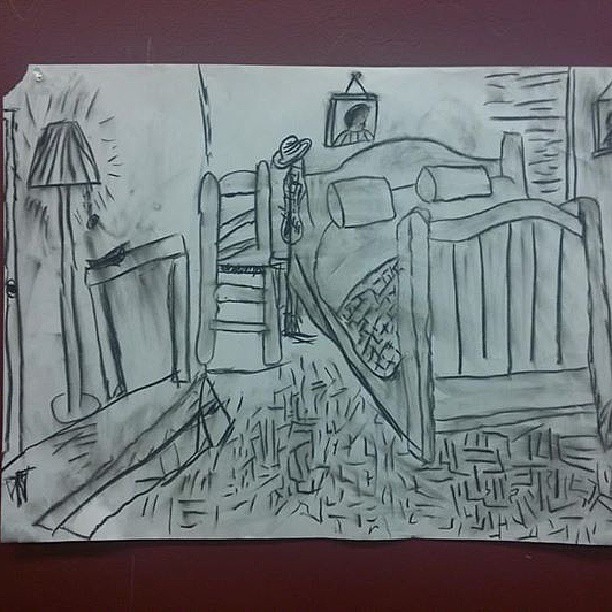This detailed pencil drawing, likely created by a child, depicts a cluttered bedroom scene. The artwork, characterized by thick lines and several smudged charcoal marks, showcases various pieces of furniture in a three-quarter perspective, all drawn on a white piece of paper with a torn top left corner. It is mounted against a brown background, possibly pinned to a dusty maroon wall. The room's elements include a wooden bed with uneven cushions and a hat hanging from its post, a crooked chair, a lamp, and a table. Additional details such as a textured floor, a rug, and two pictures—the one over the bed and another beside the bed—further enrich the scene. There is also a doorway visible, enhancing the sense of depth in this detailed, child-like sketch.